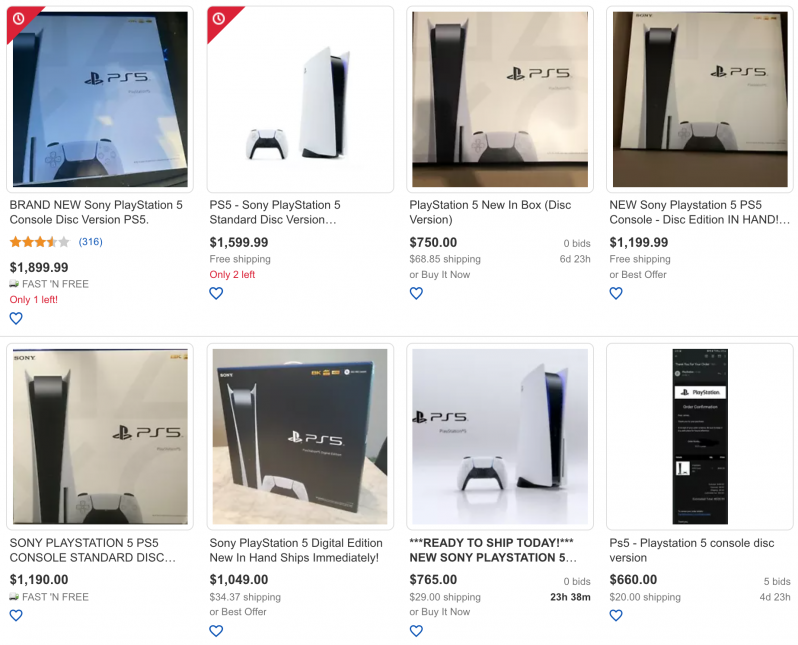Web page displaying an assortment of Sony PlayStation 5 consoles available for sale. The items are organized in two rows with four items per row, each presented in a square with a picture of the item, detailed information beneath it.

Top Row (from left to right):

1. Brand New Sony PlayStation 5 Console (Disc Version)
   - Rating: 3.75 stars from 316 reviews
   - Price: $1899.99
   - Shipping: Fast and free
   - Stock: Only 1 left

2. Sony PlayStation 5 Standard Disc Version
   - Price: $1599.99
   - Shipping: Free
   - Stock: Only 2 left

3. PS5 New in Box (Disc Version)
   - Price: $750
   - Shipping: $68.85
   - Additional Info: 0 bids, 6 days and 23 hours left for "Buy It Now"

4. New Sony PlayStation 5 Console (Disc Edition, In Hand)
   - Price: $1199.99
   - Shipping: Free or Best Offer

Bottom Row (from left to right):

5. Sony PlayStation 5 Console (Disc Version)
   - Specific details not provided in the description.

6. Sony PlayStation 5 Digital Edition
   - Specific details not provided in the description.

7. Ready to Ship Today - New Sony PlayStation 5
   - Specific details not provided in the description.

8. PS5 PlayStation 5 Console (Disc Version)
   - Specific details not provided in the description.

The webpage showcases high-demand gaming consoles with various prices, shipping options, and stock availability, giving potential buyers a range of choices.